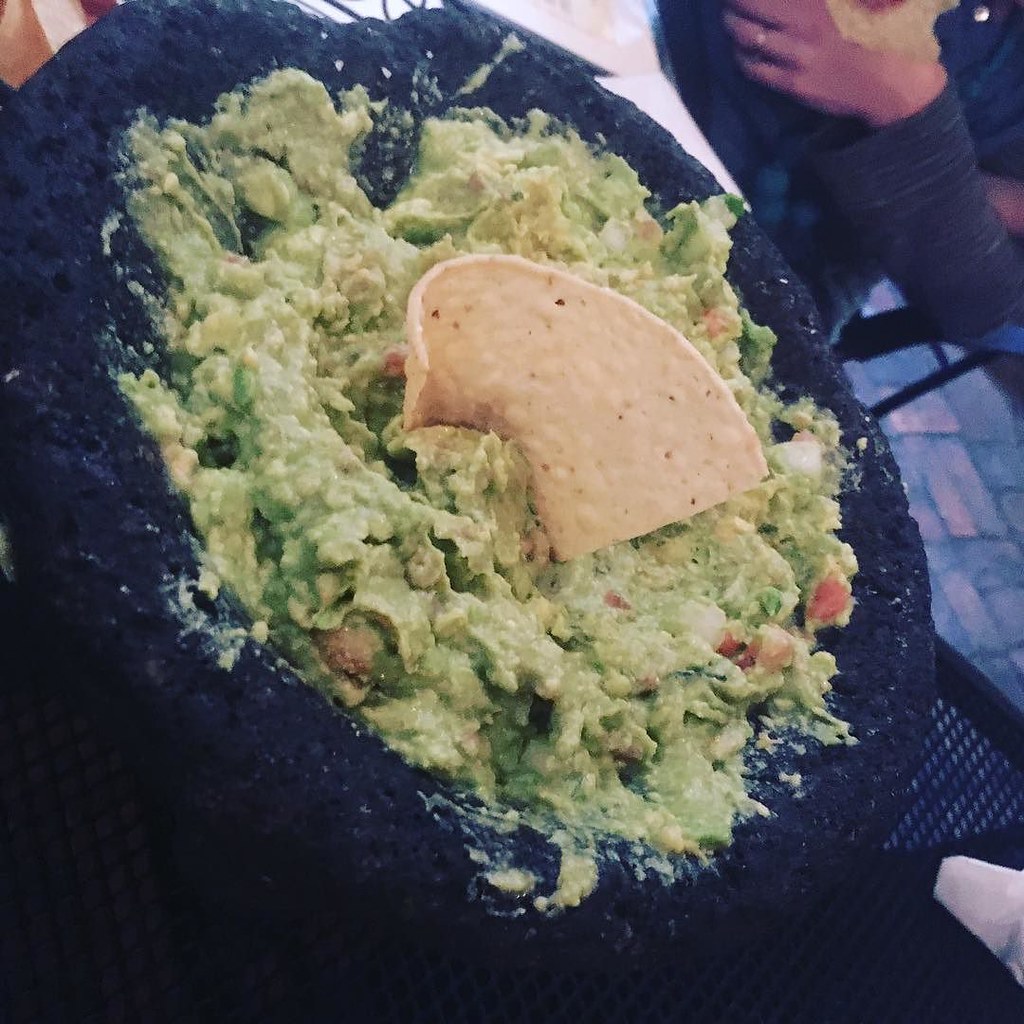This photograph captures a top-down view of a large, black stone bowl filled with freshly made guacamole, situated on what appears to be a wrought iron table with a sieve-like design. A single tortilla chip is poised in the center of the messy guacamole, ready for scooping. In the background, slightly blurred, an individual—distinguished by a wedding ring on their left hand—is seated on a chair, holding a chip. The image angle is slightly tilted, adding a dynamic element to the composition, which emphasizes the rustic and traditional vibe of the scene, reminiscent of guacamole being prepared in an authentic Mexican molcajete.